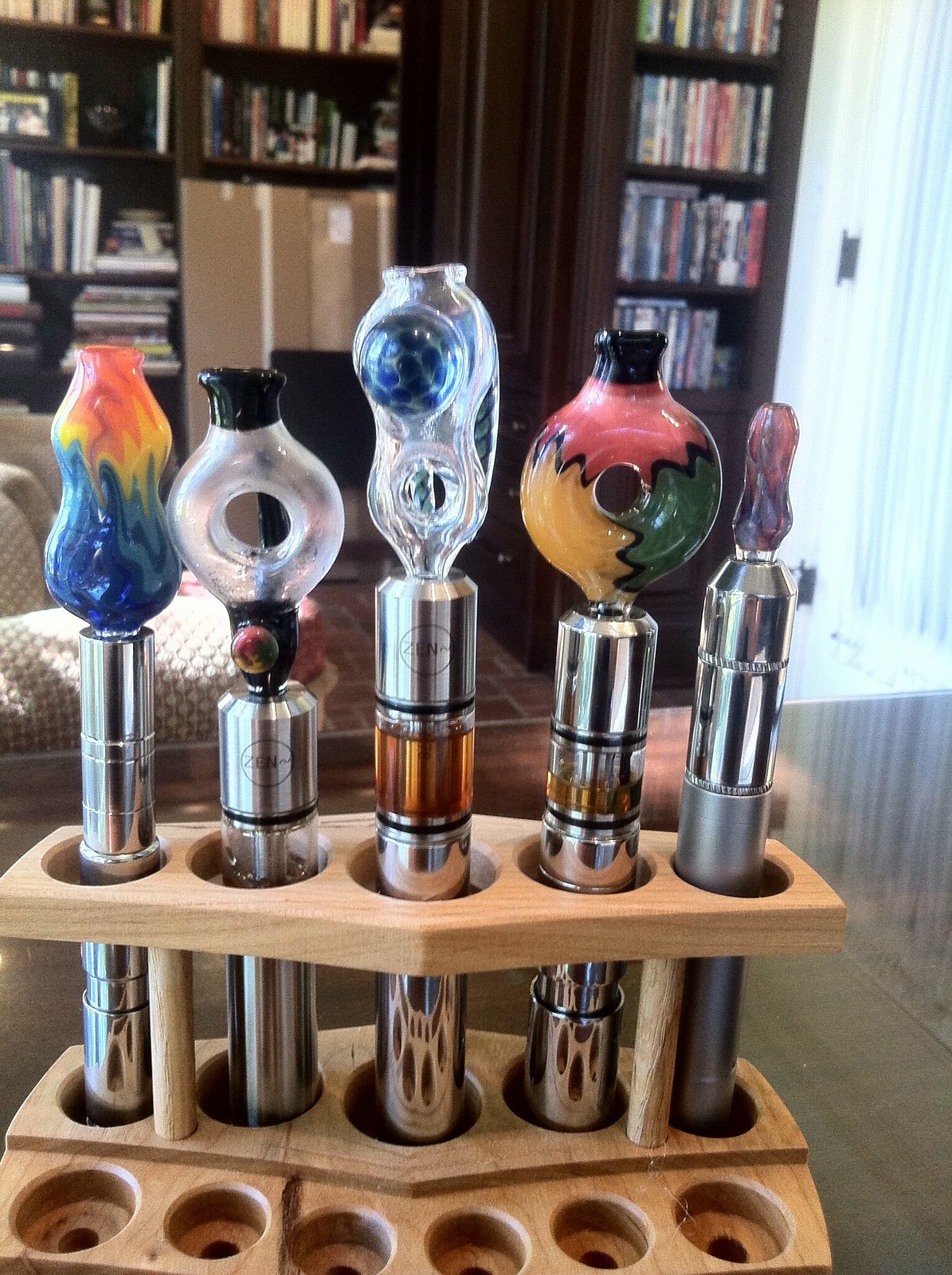A detailed colored photograph depicts an indoor scene, with a room featuring a large, packed bookshelf in the blurry background alongside some boxes, a patterned beige couch, and a possible glass door to the right. The focal point of the image is a wooden frame holding several chrome beer taps. Each tap is topped with a unique, custom-blown glass handle. The wooden holder has five metal cylindrical stems inserted into it, with additional empty holes suggesting space for more taps. Each glass handle is distinct: one resembles a multicolored, voluminous, curvy shape, almost feminine in appearance; another looks like a black and white doughnut; a third handle features a bulbous green and blue ball, giving it an alien-like look; the fourth handle is again doughnut-shaped but with vibrant yellow, red, and green colors; while the fifth and final handle has a smaller, intricate shape on top. The cylindrical stems appear to contain a brown-colored liquid, adding to the intriguing, artistic allure of the setup.